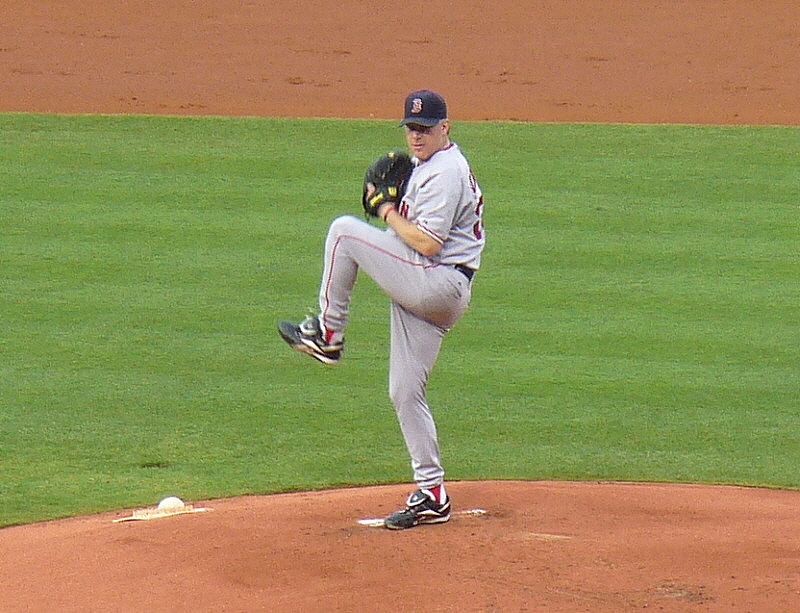The photograph captures a dynamic moment of a baseball pitcher mid-throw, deeply focused on delivering the pitch. The player is positioned on a rounded, hilly pitching mound, characterized by orange clay dirt, with a green baseball field in the background. The pitcher's uniform consists of gray pants with red stripes, a gray jersey adorned with red text, and black cleats with white and red highlights. He also sports a blue cap featuring a red logo, possibly indicating he plays for Boston. The pitcher is right-handed, as evidenced by the glove on his left hand, and his stance—with one leg lifted towards his chest—demonstrates the classic pitching form, showcasing the preparation phase of his throw. The motion is highlighted by slight blurring, suggesting the photograph was taken mid-action.